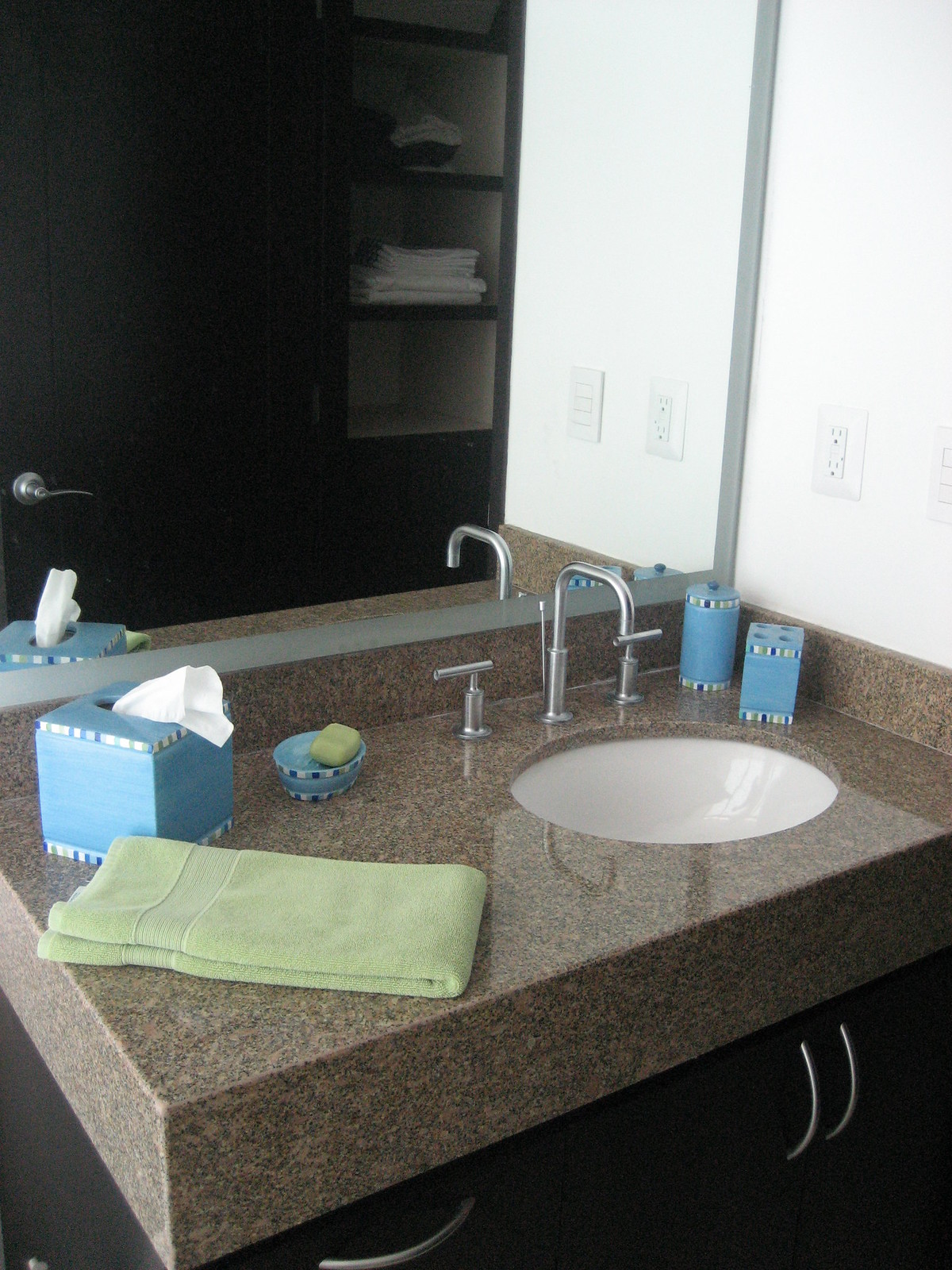This photograph captures the interior of a bathroom with a focus on a well-organized vanity area. Dominating the upper portion of the image is a large, rectangular mirror that offers a reflected view of the bathroom's opposite wall, displaying neatly folded white towels on black shelves. Beneath the mirror, a pristine granite counter extends from the upper right to the left. Central to this countertop is an elegant white sink basin fitted with a sleek, silver faucet that includes two matching handles for hot and cold water.

To the upper right on the granite surface, two blue canisters are positioned side by side—the first round, the second square—adding a splash of color. Moving leftward from the sink, there is a small blue dish holding a bar of brown soap, followed by a blue tissue box with a tissue artfully pulled out, ready for use. In the lower left corner of the counter, a light green hand towel is neatly folded.

Below the counter, part of the plumbing system is visible with two curved, silver pipes situated directly underneath the sink basin. The combination of sleek fixtures, organized toiletries, and a touch of colorful details contributes to the bathroom's polished and inviting atmosphere.